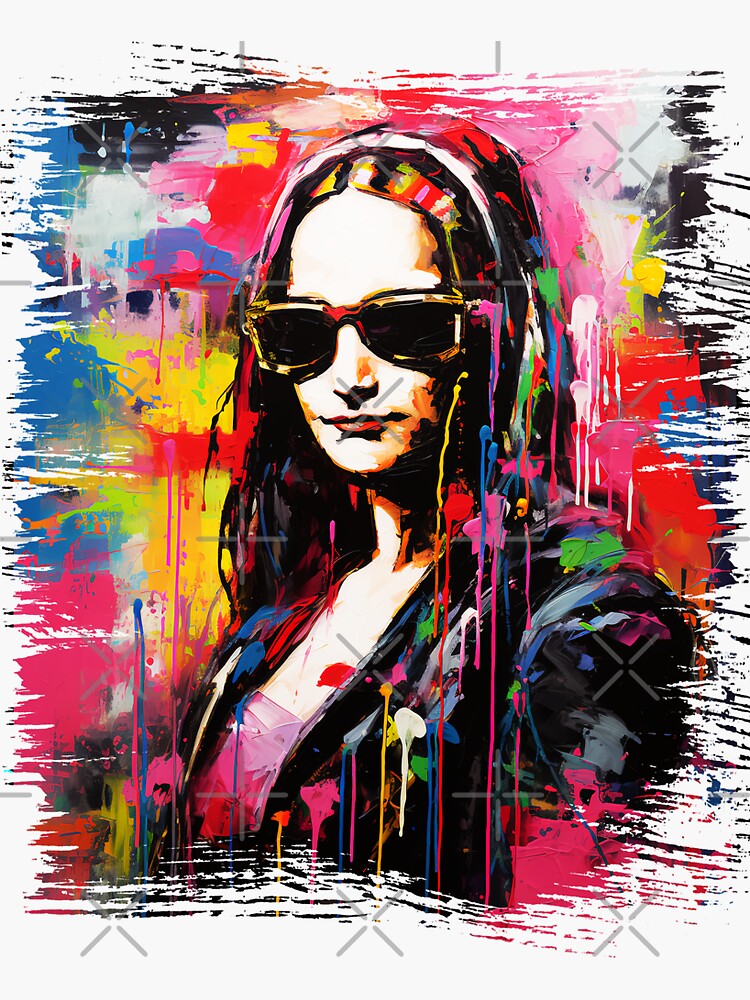This image is a vibrant, modern art interpretation of the Mona Lisa, rendered with a multitude of colors and abstract elements. The subject retains the iconic, subtle smile of the original Mona Lisa and gazes directly forward through large, dark sunglasses with gold frames. Her long, dark hair is streaked with colorful paint that drips down, adding a dynamic feel to the composition. She wears what seems to be a black leather jacket splattered with varied colors over a pink shirt, revealing a plunging neckline.

The background is a kaleidoscope of watercolor hues—red, pink, orange, blue, yellow—applied in an intentionally chaotic manner, with paint splotches and drips that give a sense of movement. Black and white lines frame the top, left side, and bottom of the painting. The artistic chaos is echoed by multiple watermark X's across the image to deter unauthorized use.

The woman also sports a red hood with a white tip, which covers part of her head and adds more layers to her modern, slightly rebellious appearance. Her serene expression is punctuated by red lipstick, and some paint even trickles down from the ears but avoids her face, emphasizing the abstract and spontaneous nature of the artwork. Despite—or perhaps because of—these modern and abstract touches, she remains distinctly recognizable as the Mona Lisa, transformed into a contemporary icon bursting with color and style.